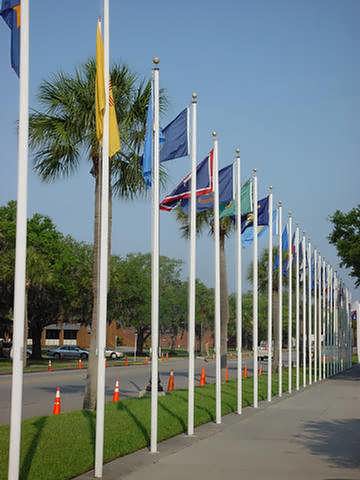The photograph captures a wide sidewalk adorned with many white flagpoles, each crowned with a silver ball and hoisting colorful flags, possibly representing various states or countries. The flagpoles, aligned in a neat row, are slightly shorter than the surrounding palm trees that are also planted along the sidewalk. A shadow of a tree falls across the pavement, enhancing the outdoor scene under a clear blue sky. Across the street, a row of trees partially conceals a brick building. Orange traffic cones line both sides of the road, which has parked cars and a truck progressing down it. The sidewalk gives way to a strip of grass between the flagpoles and the road, where more trees can be seen running parallel to the flagpoles, suggesting the possible preparation for an event like a parade.